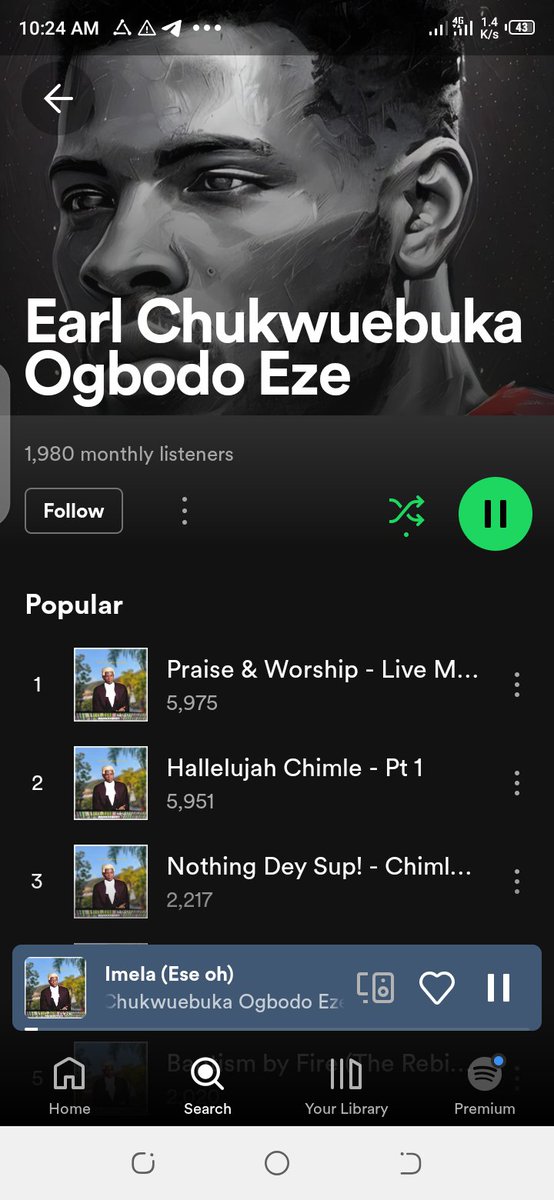This image is a screenshot of a Spotify page for the artist Earl Chukwubuka Ogbodo Eze. The artist's name is displayed prominently, with 1,980 monthly listeners indicated beneath it. The page features a "Follow" button enclosed in a rectangular box, adjacent to three dots for additional options. Below, there are green "Shuffle" and "Pause" buttons, maintaining Spotify's iconic color scheme.

The section titled "Popular" lists the artist's top songs. The titles include "Praise and Worship Live" (truncated with "m..."), "Hallelujah Chimley - Pt. 1," and "Nothing Day Sup - Chiml...," suggesting longer names that are cut off. One song is currently playing, only partially visible with the letters "l-m-e-l-a" followed by "(ESE OH)" in parentheses, indicating the track has recently started.

At the bottom, the navigation bar includes "Home," "Search," "Your Library," and "Premium," the latter marked by a blue dot, indicating a highlighted or selected state. Below these options, the Android device's navigation buttons are visible, and the time shown is 10:24 a.m., marking when the screenshot was taken. The entire layout is characteristic of the Spotify app's interface on an Android device.